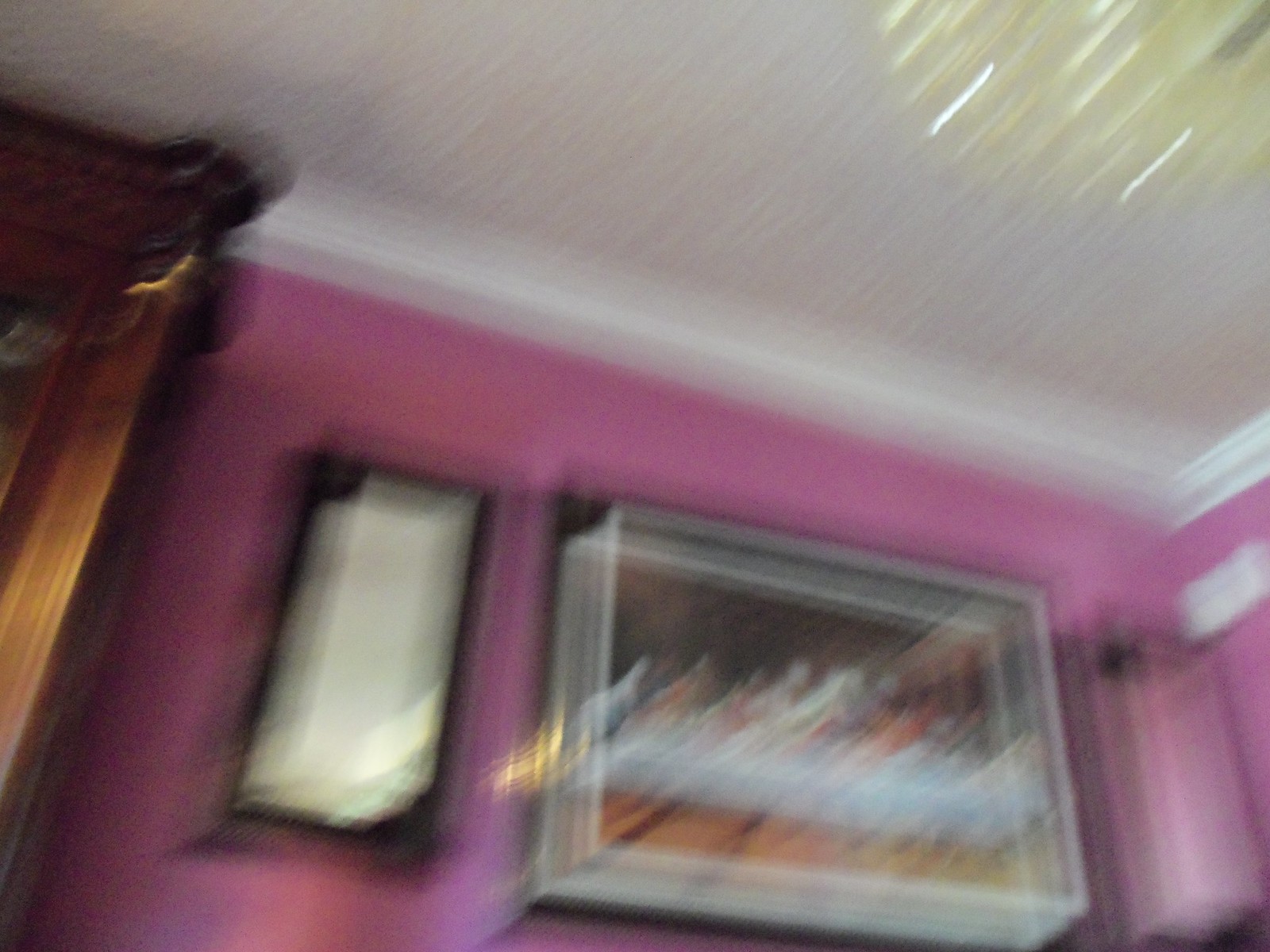This is a photograph taken indoors, likely within a brightly-colored living room or similar space, capturing a scene with significant motion blur. The walls are painted a striking orchid pink, augmented by a sophisticated white trim along a tan ceiling. Central to the image is a framed painting of the Last Supper, encased in what appears to be glass, which seems to jut out from the wall. This religious artwork forms the focal point of the photo, though its details are marred by the blur. To the left of it, there is another vertical, tan-colored piece of artwork framed in black, though its contents are indistinguishable due to the photo's quality.

Also visible in the image's left-hand side is the corner of an ornate, dark wooden cabinet, largely cut off in the photo. In the upper-right corner of the image, there is a round, crystal-like light fixture, adding a luxurious touch despite its appearance of being in motion. Overall, the room exudes a blend of opulence and vibrant color, though the photographic blur obscures finer details.